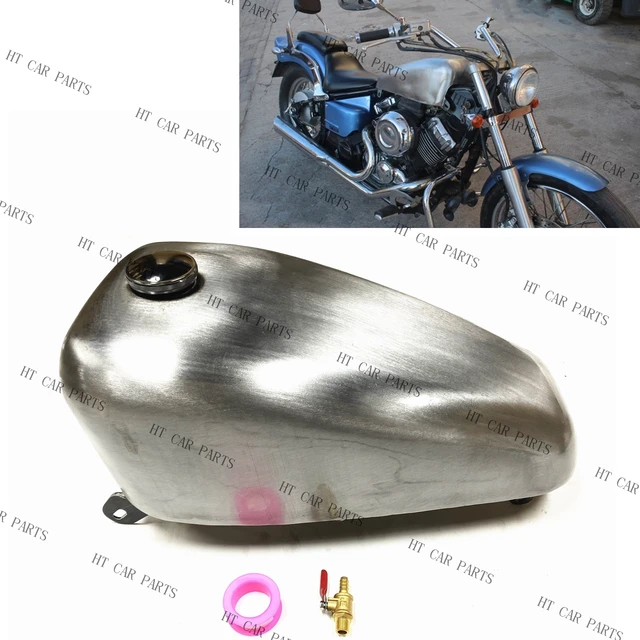The image features a composite advertisement for HT Car Parts, showcasing multiple photographic elements set against a white background, which is diagonally overlaid with four repeating stripes of the text "HT Car Parts" in gray. The primary focus is a slightly older, blue-highlighted motorcycle with a silver gas tank and thin handlebars, parked on dark gray pavement without a rider. Below the motorcycle is a polished silver gas tank displayed separately, with its fuel cap facing the opposite direction. Additionally, the image includes two small parts: a pink O-ring and a gold valve with a metal rod tipped in red. These elements, possibly enhancements or replacements for the motorcycle, are featured prominently to highlight the parts offered by HT Car Parts.